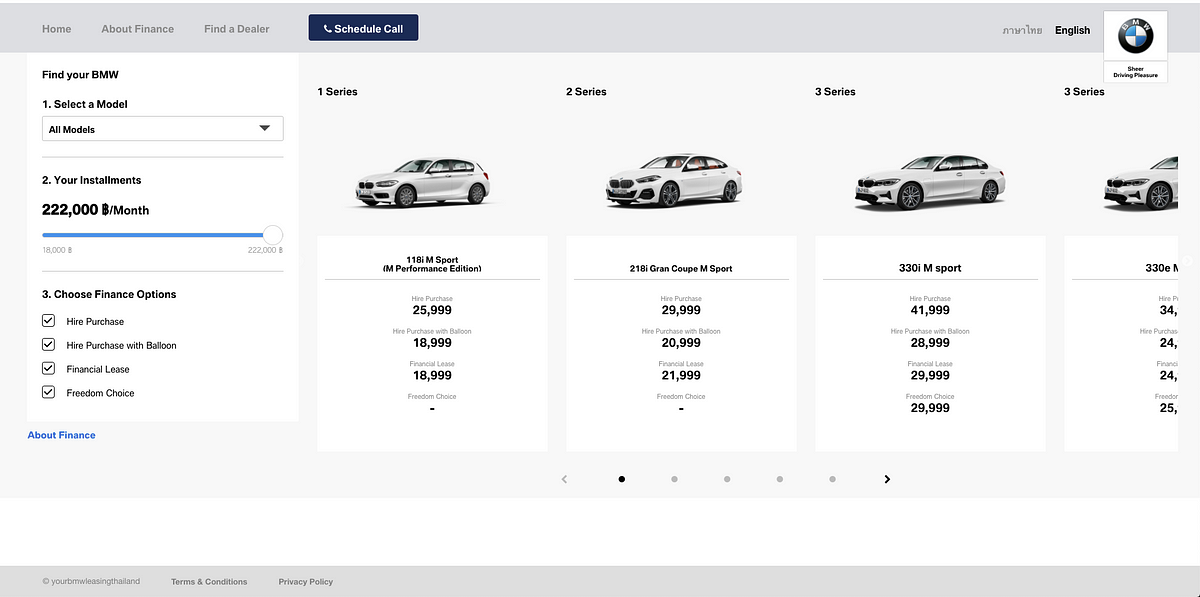Screen capture from a BMW webpage displaying a filtered search page for selecting a vehicle. On the left side, there is a column of filters to tailor the search. The first filter is a drop-down menu labeled "Select a Model," listing all available BMW models. Below that, there is a slider bar for "Installments," allowing the user to adjust their desired monthly payment amount. The last filter section includes three financing options: "Higher Price," "Higher Price with Balloon," "Finance," "Lease," and "Freedom Choice," each with a corresponding checkbox.

On the right side, there are three images showcasing different BMW vehicles with three-quarter views, highlighting the front-left and left sides of the cars. The first car displayed is a BMW Series 1, and below each vehicle image, there are detailed specifications and associated finance options, though the text is too small to read clearly. The car images are arranged in a row from Series 1 to Series 3 and beyond.